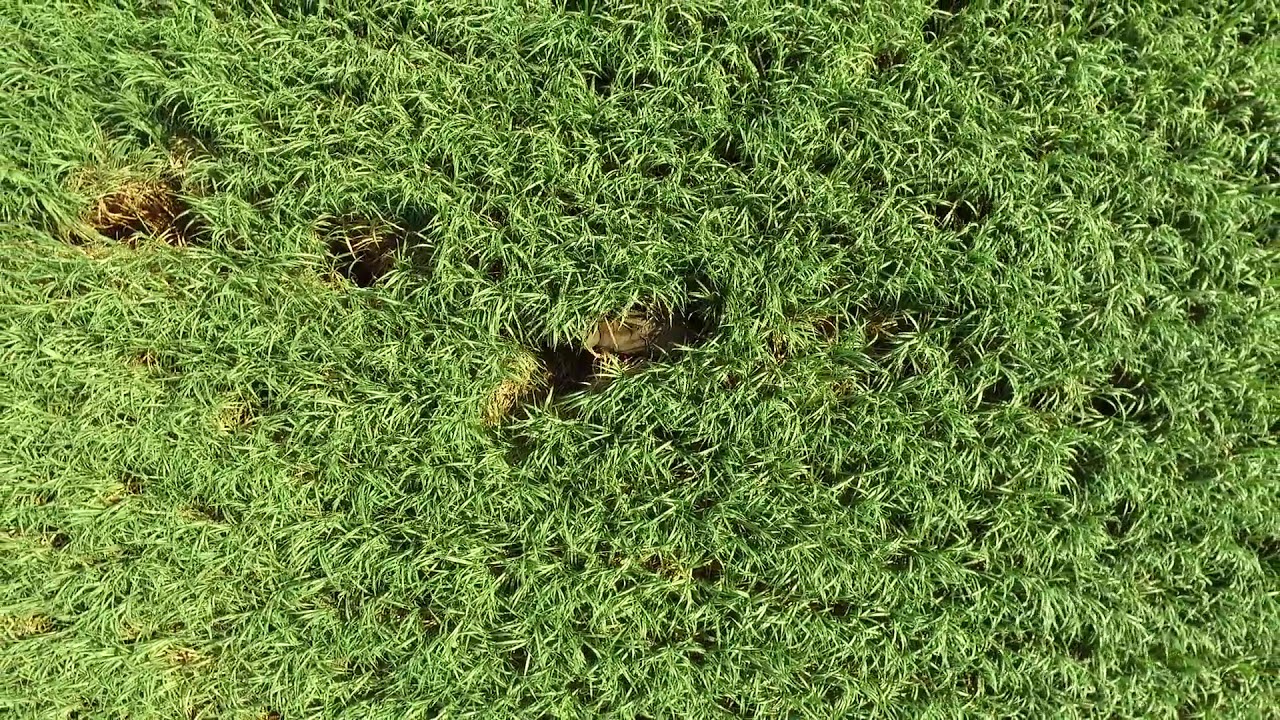This aerial photograph captures a horizontal rectangular view of a lush, green grassy area, resembling a mossy ground from above. The entire frame is densely covered with plush grass or moss, with a gradient of colors transitioning from a lighter yellowish-green on the left to a darker bluish-green on the right. Scattered across this verdant landscape are a series of indentations or gouges, which may be footprints, hoof prints, burrows, or simply empty holes. 

In the upper left corner, a nearly round indentation is visible, with another similar one just to its right. The center of the image features a more prominent and oblong-shaped depression. Additionally, towards the lower right corner, areas of the grass exhibit a gradation towards a yellowish hue. The detailed texture of the blades is apparent, offering a sense of the grass's height and density. There is no text or human presence in the image, emphasizing the natural, undisturbed quality of the scene.